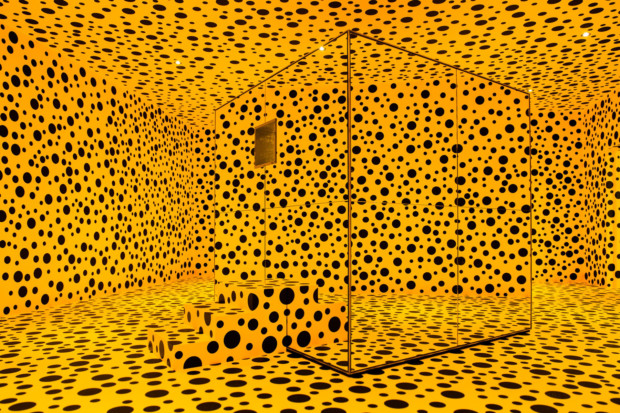The image depicts an optical illusion created within a large, square room predominantly colored in varying shades of yellowish-orange, with a more intense orange hue concentrated at the corners. The entire space, including the floor, walls, and ceiling, is covered in an array of black polka dots of different sizes scattered in a haphazard pattern, adding to the visual complexity. At the center of the room stands a three-dimensional mirrored cube, outlined by darker black lines, which reflects its surroundings, further enhancing the illusion. On the left side of the cube, there are three yellow steps adorned with the same random black polka dots, leading up to a window or viewport into the interior of the mirrored structure, creating a mirror image effect and enriching the overall surreal experience of the scene.